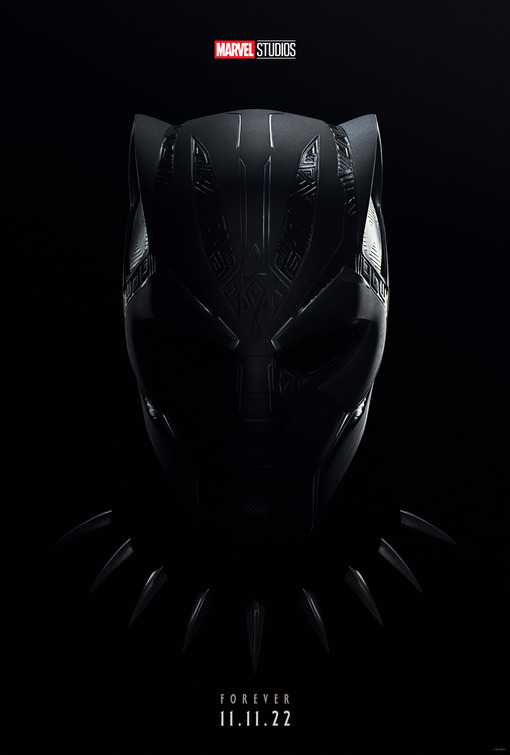This image is a movie poster for Marvel Studios' "Black Panther." At the very top, it features the "Marvel Studios" logo in striking red with a white border and black outline. Dominating the center of the poster is the striking silhouette of the Black Panther mask, characterized by its distinct cat ears and subtle eye contours. The mask is accompanied by the iconic Black Panther necklace, adorned with teeth or claws around the neck, creating a powerful visual. The background is pitch black, making the mask and necklace stand out, and there is some light illuminating the mask, adding to its dramatic effect. Towards the bottom, the poster displays the text "Forever" alongside the release date "11.11.22," possibly as a tribute to the character or the actor. This modern and sleek design captures the essence of the film.